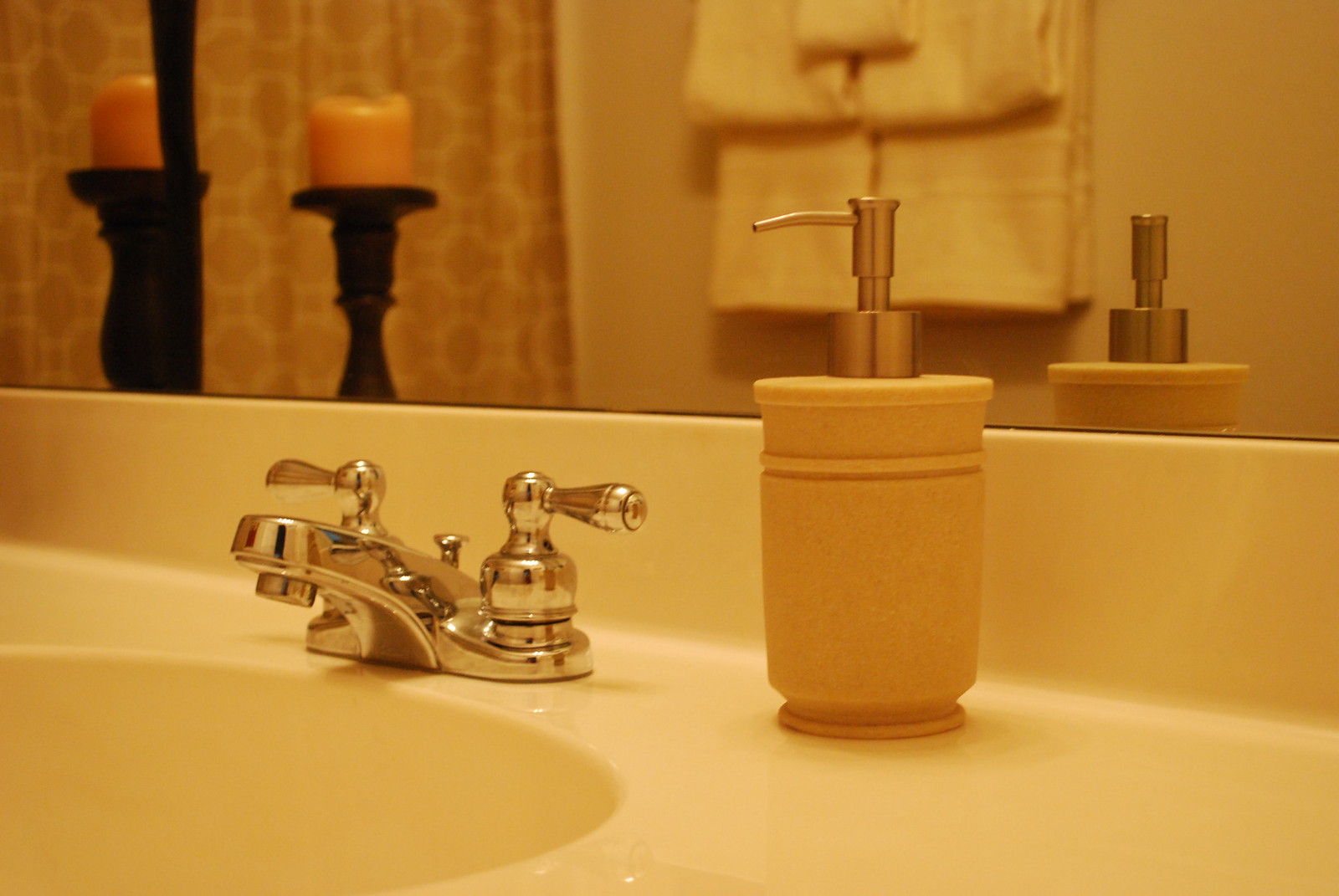The image depicts a well-appointed bathroom with a large mirror spanning the upper wall. Below the mirror, a brown wooden door is visible. The room features two black candlesticks, each holding a sizable yellow candle, which form a striking contrast against the light yellow walls. Hanging on a rack, there's an organized set of towels: two large, two small, and a washcloth.

The sink area includes a light yellow countertop paired with a shiny, ornate gold faucet equipped with traditional turn nozzles. The sink is oval-shaped, smoothly integrated with the countertop. A glass soap dispenser, designed with a rounded base and barrel-like midsection, is placed on the counter. It has a decorative indented circle near the top and is topped with a gleaming gold dispenser.